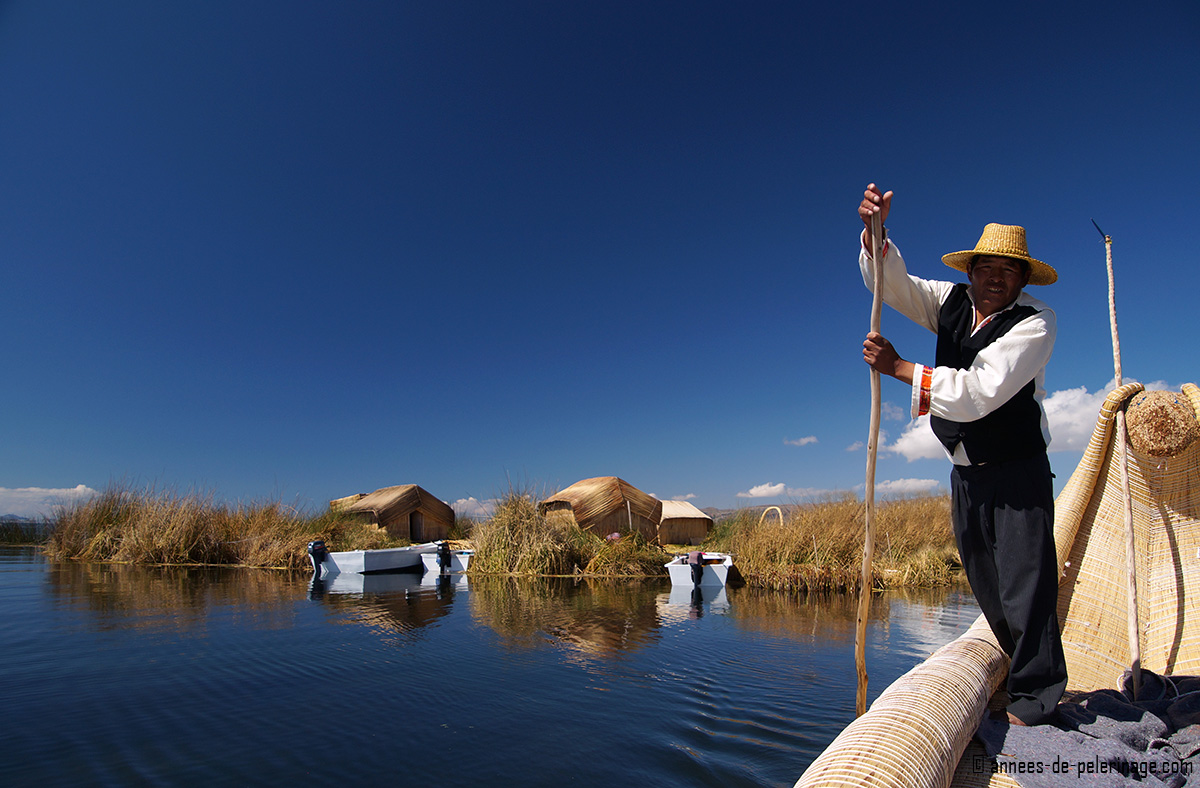In this photograph, a middle-aged man with brown skin is skillfully navigating a traditional gondola-like boat across calm waters. The man, likely Peruvian, is standing at the front of the boat, clad in a black vest, loose black pants, a white long-sleeve shirt, and a distinctive cowboy or strong hat. He grips a long wooden stick, using it to propel the boat forward. The gondola itself appears to be crafted from light wood or fabric, and it features intricate details with white strings atop it, adding to its handmade appearance. The back of the boat curves high into the air, and a partially visible foreign word adorns the bottom right corner. The serene backdrop reveals a floating village characterized by small white motorboats docked along a reed-filled shoreline. Beyond the reeds, a few handmade huts constructed from reeds or wood can be seen. The tranquil scene is set under a mostly clear, vibrant blue sky with just a few clouds near the horizon, illuminating the picturesque marshland.